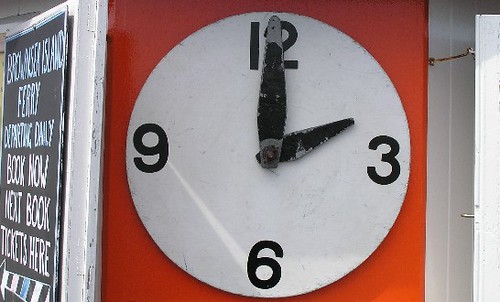A photograph showcasing a clock mounted on the side of a business building. On the left side of the image, a white door is prominently featured against the white exterior wall of the building. To the right, there is a black sign with multicolored font, featuring both bluish and white text, which appears to be advertising ferry services with visible inscriptions such as "Book Now" and "Book Tickets Here," accompanied by an arrow. The clock itself is centrally located between the sign and the door, displaying a white clock face with partially peeling black hands and visible numerals at the 12, 3, 6, and 9 positions. The white clock face stands out against a vibrant red-orange background.